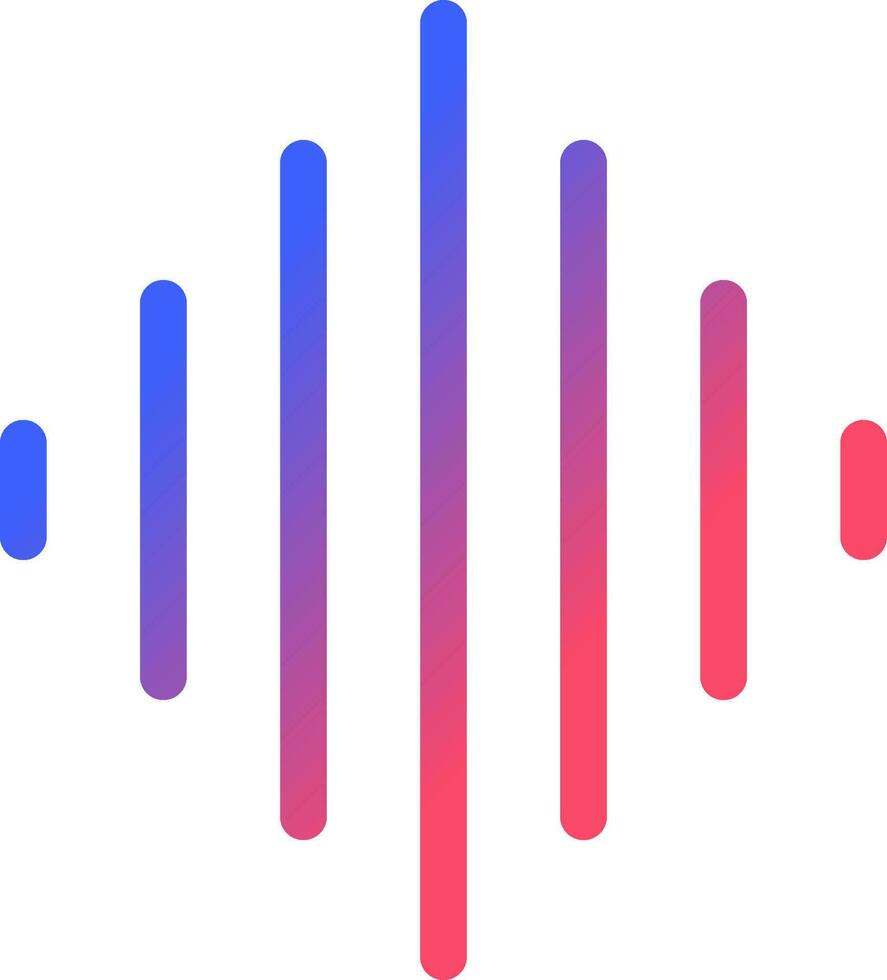A square image featuring a symmetrical series of seven vertical lines on a white background. From left to right, these lines progressively transition in color from blue to purple to red, capturing a gradient spectrum. The central line is the longest, creating a visual peak in the middle of the image, while the lines on either side decrease in height, forming a diamond-like shape. The color transition begins with a short blue line on the far left, moving through various shades of purple in the middle, and culminates with a short red line on the far right. The image evokes the appearance of a sound frequency spectrum or a music analyzer display, suggesting a connection to audio visualization.